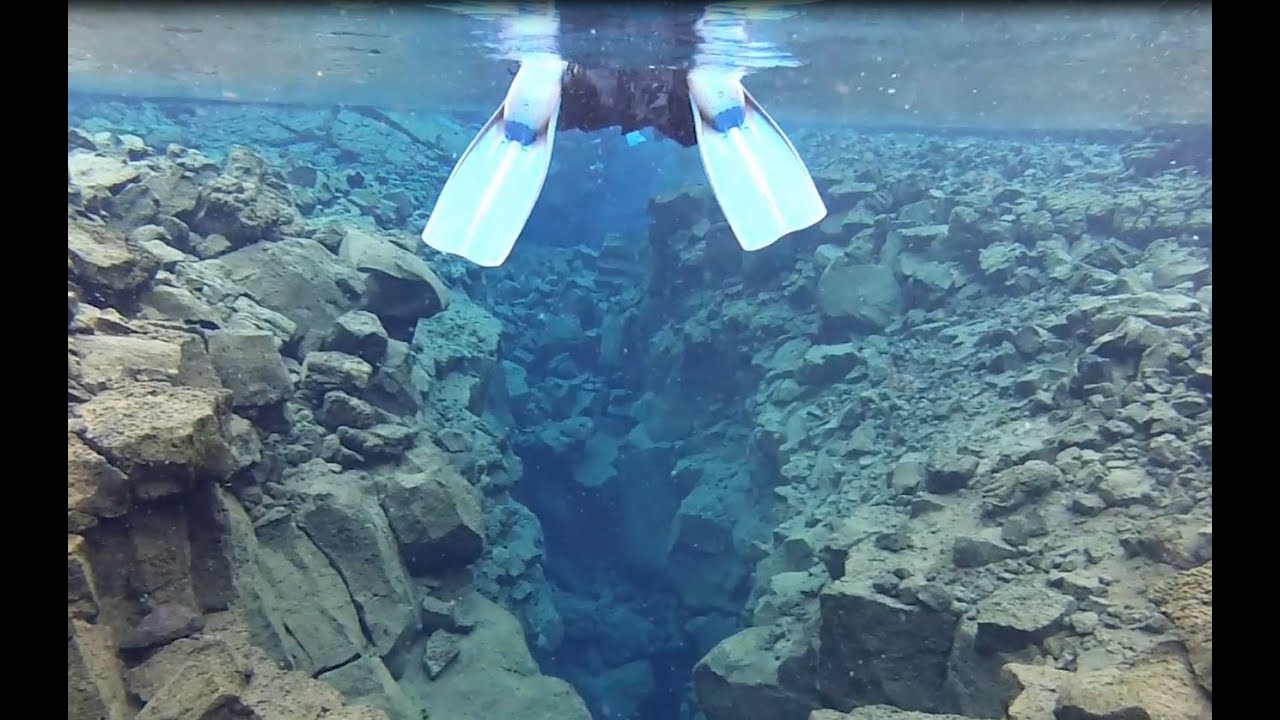This underwater scene showcases a diver adorned with black fins and a likely black diving suit. The clear, blue-green water reveals an underwater canyon or valley filled with medium to small-sized rocks, devoid of any fish, plants, or other organisms. The diver's body and face are not visible; only the back of the flippers can be seen as they swim just below the surface. The tranquil setting, with its distinct underwater hue, highlights the stark, lifeless landscape of rocks beneath the diver. The shallow depth of the water, estimated to be around 20 to 30 feet, adds to the clarity and visibility of the scene.